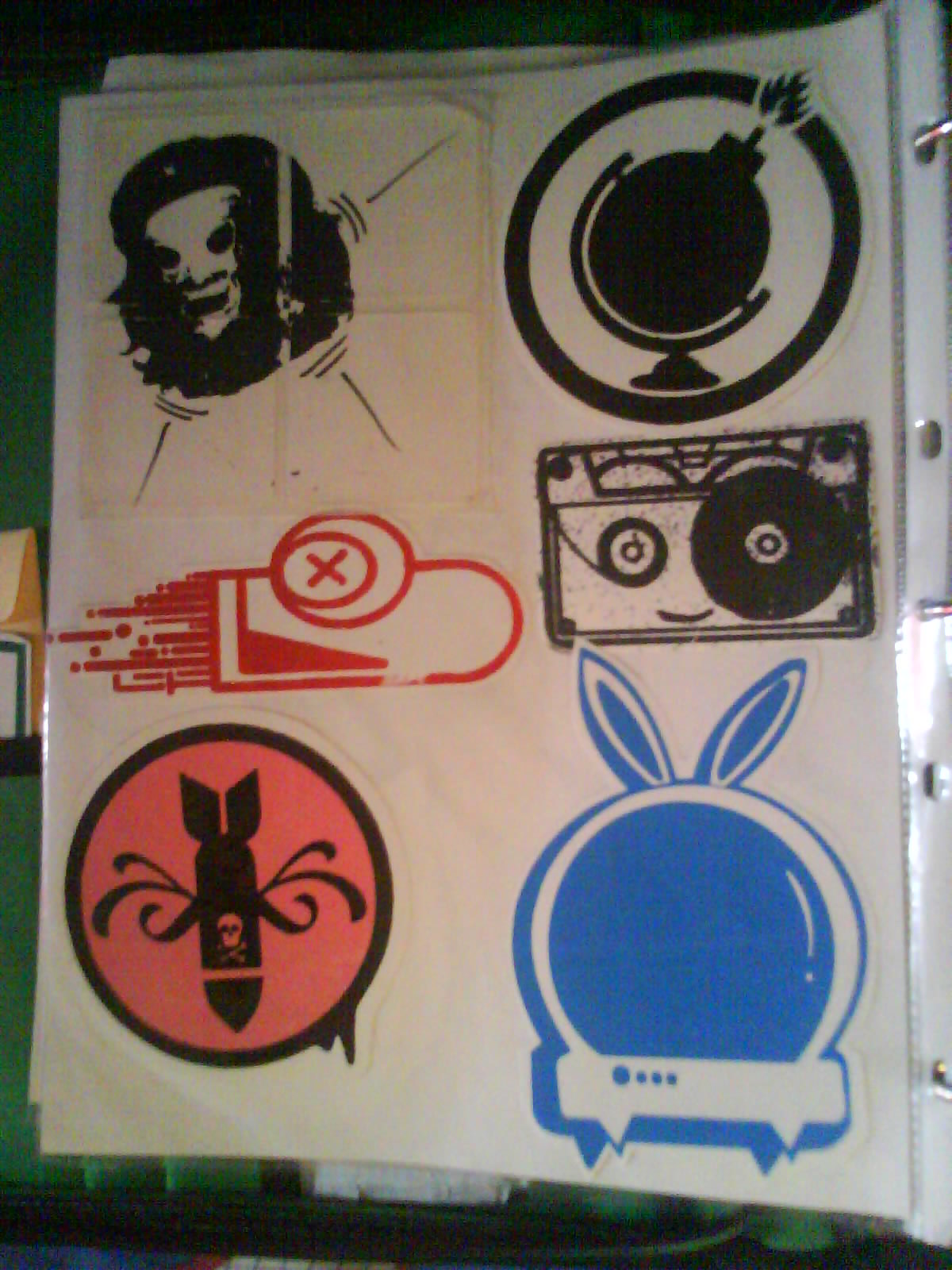The image depicts a white A4-sized sheet, likely within a plastic compartment of a three-ring binder, as suggested by the visible metal rings on the right edge. This sheet appears to showcase various stencil designs in vibrant colors. In the top left corner, there's a stencil resembling Che Guevara with simplified eyes. Adjacent to this, on the top right, is an image of a bomb integrated into a globe, complete with a lit fuse. Further down, aligned below this on the right, is a black cassette tape. On the left side, there's a design with a red line and another of a bomb with flames, featuring a skull at the center. Finally, in the bottom right corner, there’s a blue, circular cartoon-like image, possibly of a TV, adorned with blue bunny ears and white accents for reflection.